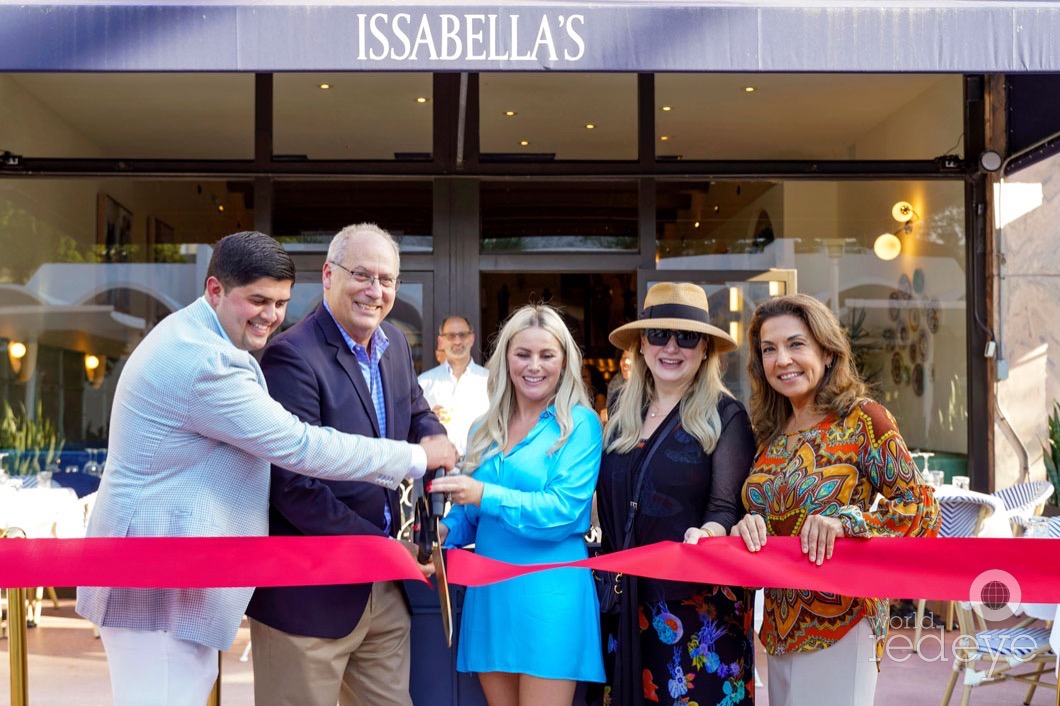In front of the classy and sophisticated establishment called Isabella's, identifiable by its name in white font on a light gray awning, a ribbon-cutting ceremony is taking place. The storefront features glass doors and windows, all closed, accentuating a sleek and modern design. Six individuals, all Caucasian Americans, are gathered in the forefront, smiling and engaged in the ceremony. The central figure, a blonde woman in a light blue long sleeve dress, is cutting the bright red ribbon with an oversized pair of scissors, opening the establishment. She is flanked by two men on her left: one in a blue suit and another in a gray blazer with khaki pants and a plaid shirt. To her right, two women aid in holding the ribbon: one in a black sweater and another in a floral and sheer dress, accessorized with sunglasses, a hat, and a purse strap. The mood is celebratory and welcoming, heralding the opening of what appears to be a sophisticated new restaurant. In the lower right corner of the image, the logo "World Red Eye" is visible.